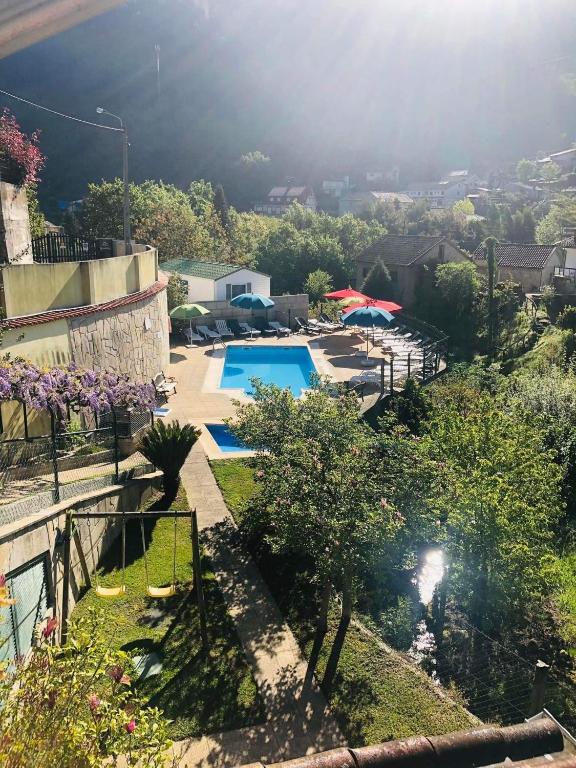The vivid color photograph captures a picturesque hillside home with a sprawling backyard that features a rectangular swimming pool, encircled by vibrant sun parasols and lounge chairs. In the foreground, a delightful garden area holds a swing set for children, connected to the pool by a well-defined walking path. This path further ascends a gently sloped hill adorned with arched flower arbors, their purple blossoms forming a natural canopy. A black chain-link fence outlines the sloped walkway on the left, while on the right, fencing marks the yard's boundary. A large, rounded stone wall accents the pool area to the left. The image showcases a lush, tree-filled residential landscape, with homes dotting the hills and the sun casting a gentle glow, adding a serene yet vibrant atmosphere to the scene.